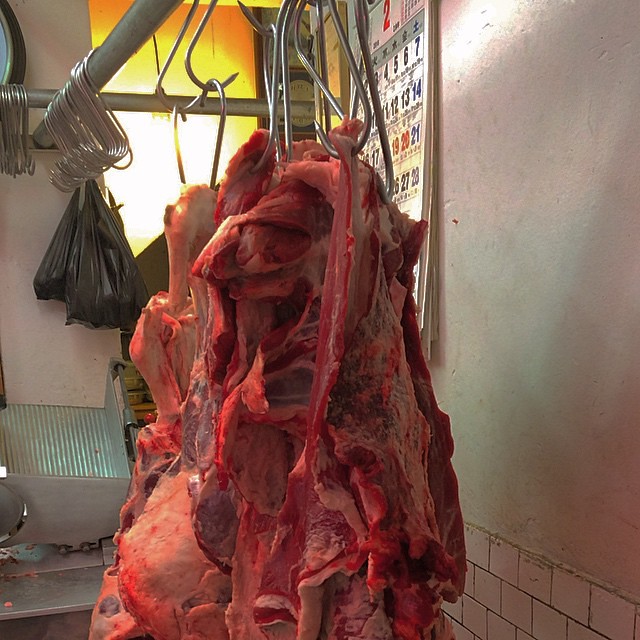The photograph depicts the interior of a butcher shop, highlighting a large, freshly butchered slab of meat hanging from metal hooks attached to a metal rod. The meat appears bright red, indicating it was likely slaughtered recently. Nearby, additional hooks hold at least two black plastic bags, their contents indeterminate. The background reveals a white wall partially covered with a calendar, showing the number "2" in red and dates up to the 28th, though much of it is obscured by the hanging meat. Below the calendar, there are white ceramic tiles lining the lower portion of the wall. On the left side of the image, a meat slicer machine is partly visible. Scattered pieces of meat are seen on a silver table in the background, adding to the detailed, slightly eerie atmosphere of the scene.